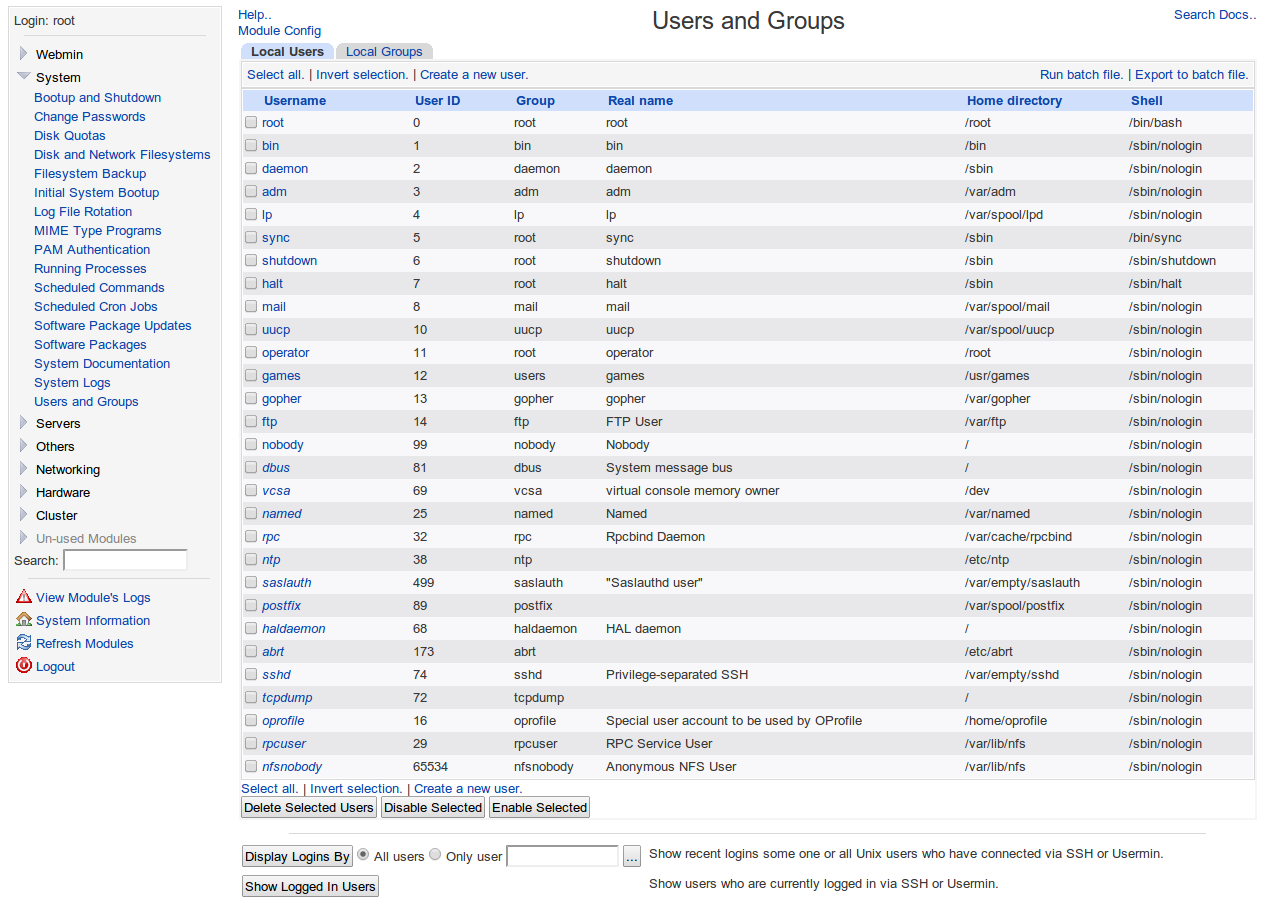The webpage displays a detailed list of users and groups in a system administrator interface. On the left side, there are menu options listed including "Login," "Root," "Web Administrator," and "Systems." The main content on the right side, under the heading "Module Confirmation," shows categorized sections for users and groups. Specifically, the "Local Users" section is prominent, listing details across columns such as "Username," "User ID," "Group," "Real Name," "Home Directory," and "Shell."

The user list includes entries for usernames such as "root," "ben," "Damien," "ADM," "LP," "sync," "shutdown," "halt," "mail," "UUCP," "operator," "games," "gopher," "nobody," "dbus," "VCSA," "named," "RPC," "RFP," "SAS," "IA," "ATH," and many more, totaling 30 entries. Each user is associated with a user ID and a respective group, with "VCSA" noted as one of the larger entities. This detailed display provides an exhaustive overview useful for system administration.